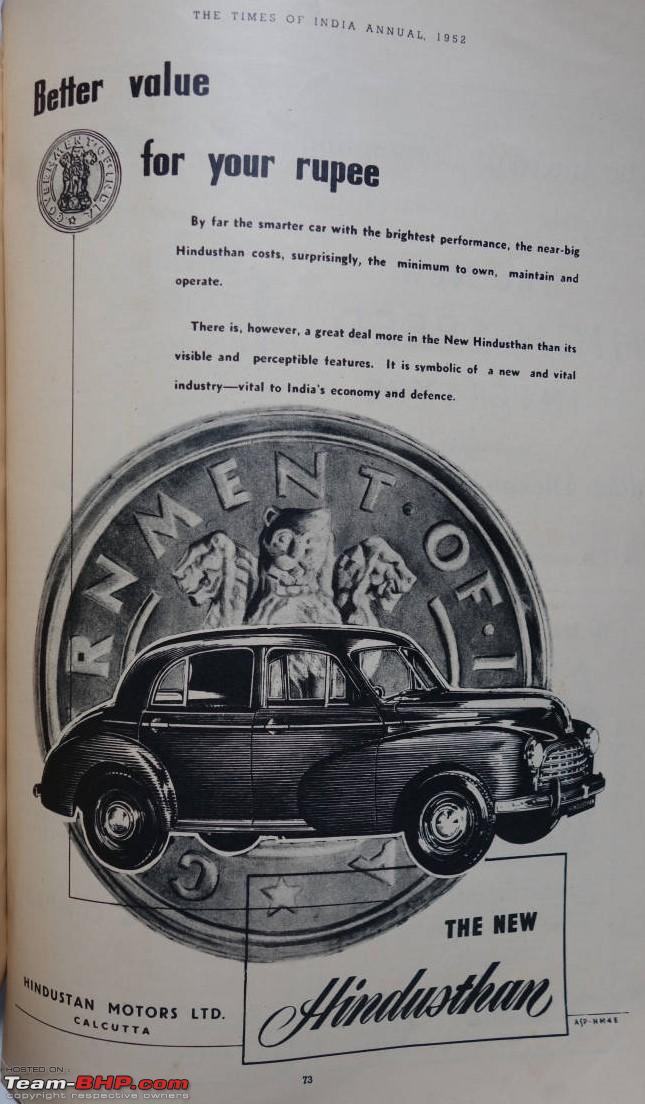The image is a detailed black-and-white magazine advertisement for the new Hindustan car, circa 1952. The page is dominated by a heading that reads "The Times of India Annual 1952" at the very top. Centered prominently on the white background is text in bold that states, "Better value for your rupee." Beneath this, in smaller lettering, it declares, "By far the smarter car with the brightest performance. The near big Hindustan costs surprisingly the minimum to own, maintain, and operate. There is, however, a great deal more in the new Hindustan than its visible and perceptible features. It is symbolic of a new and vital industry, vital to India's economy and defense."

At the center of the page, there is an intricate black ink drawing of an old-fashioned, four-door car, reminiscent of the 1940s. Placed behind the car is a large coin displaying three lion heads and partially legible text that likely reads "Government of India." Below the illustration, the ad prominently features the vehicle's name in large text: "The New Hindusthan," with a line underneath and enclosed within a box. Further down, the text "Hindustan Motors Limited, Calcutta" is visible. A circular logo of the car company, set apart from the text, includes an image of the vehicle above it. The advertisement includes a webpage watermark, "team-bhp.com copyright respective owners," indicating the image's current digital ownership. There is also a page number, likely 13, at the bottom of the page.